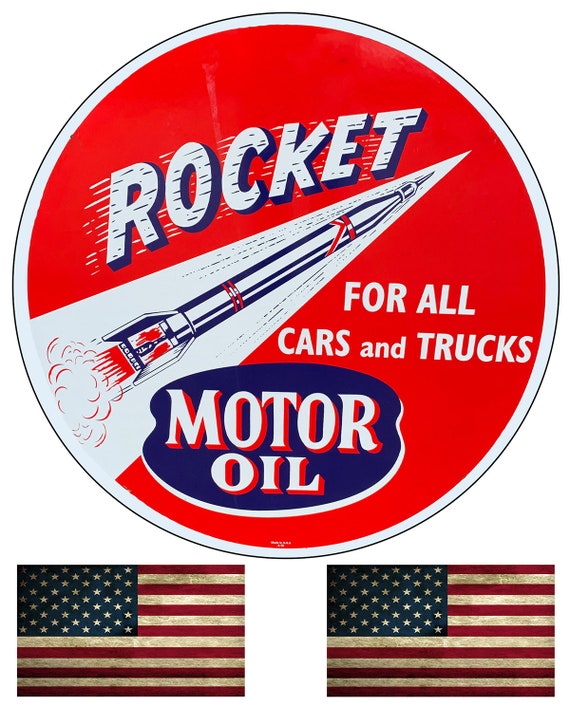This is an American advertisement for Rocket Motor Oil, designed with a patriotic theme. At the center of the image is a large, vintage-style circular logo outlined in black, followed by a gray inner border, and a red background. Within the red circle, a white area resembles a large slice taken out, creating a dynamic visual slice effect. Across this white section is an illustration of a blue rocket decorated with red bars and emitting red flames with red smoke lines, emphasizing speed and power. The word "Rocket" is prominently displayed in blue and white letters with speed lines, accentuating motion, while "Motor Oil" is written in white letters with a red shadow, set against an oval shape with a blue background.

The slogan "For All Cars and Trucks" is featured in white text within the red part of the logo. At the bottom of the advertisement, two identical American flags are positioned on the left and right sides, appearing worn and slightly dirty, enhancing the vintage appeal. The overall design echoes a nostalgic, patriotic theme with a palette limited to red, white, and blue, encapsulating the spirit of American automotive culture.